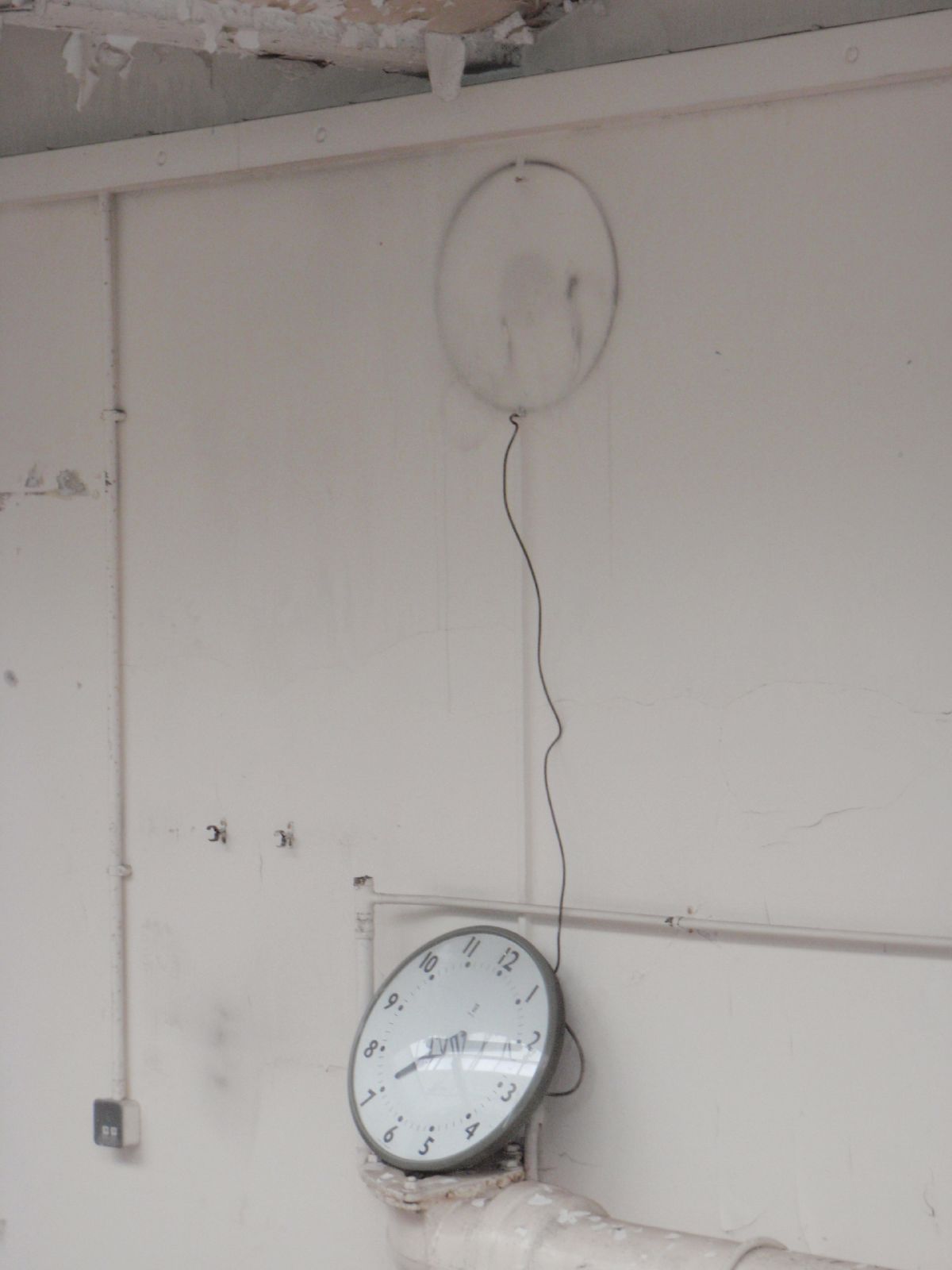This portrait-style image depicts a dimly lit, white plaster wall with visible signs of aging and damage, particularly a cracked and ripped ceiling exposing insulation and dry wallpaper. A round clock with a dark gray case, a white face, and black numbers and hands, which reads 7:11, has fallen and is now resting on a prominent white metal water pipe. The clock was originally affixed to the wall, leaving a bold, dirty circle imprint where it once hung. A wire still connects the back of the clock to its original hanging spot. To the left of the clock, there's an electrical outlet attached to the wall. The overall setting suggests a basement or a similar space with some exposed electrical wiring and an aged, slightly dirty ambiance.